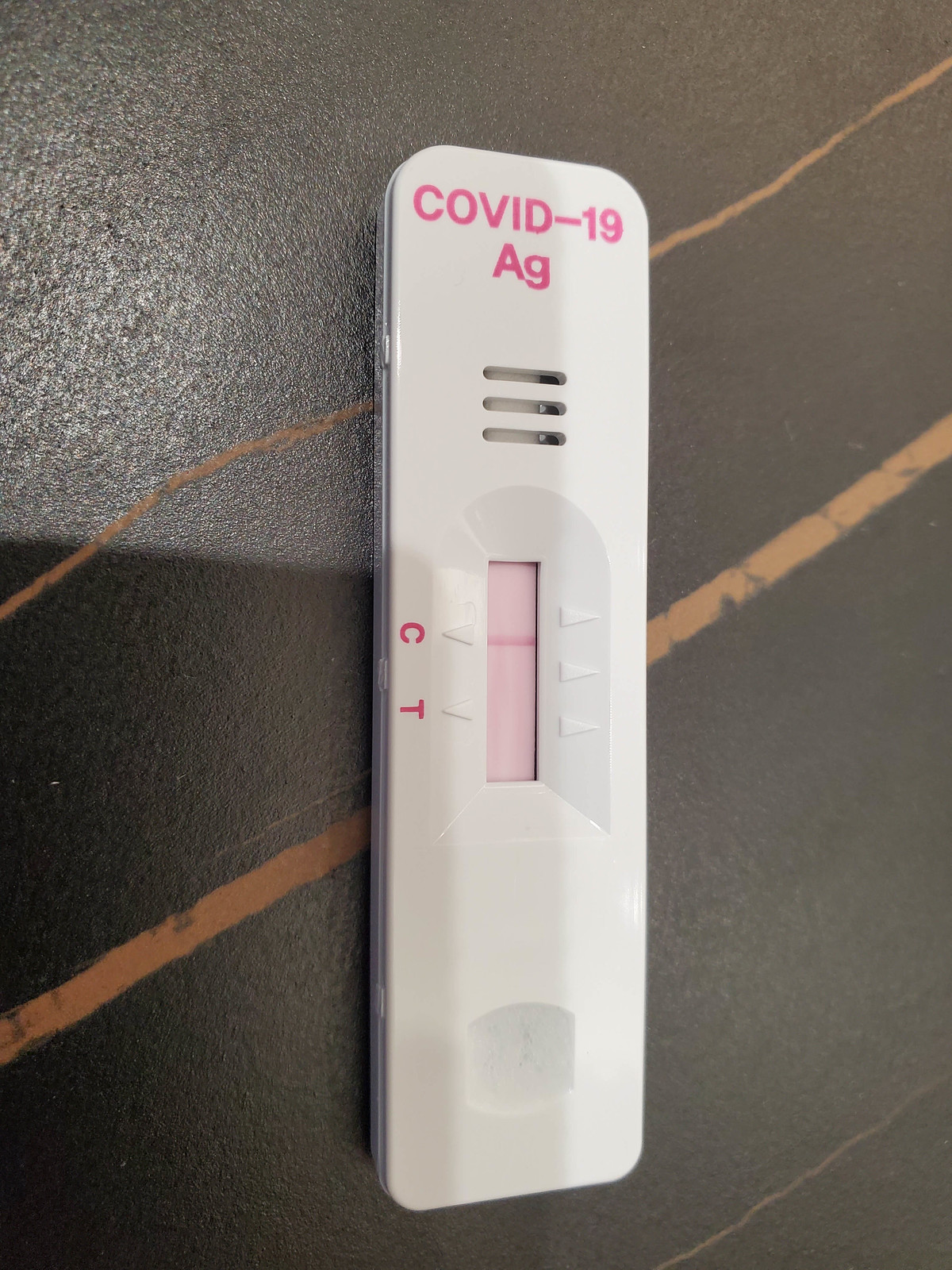This detailed photograph captures a COVID-19 test resting on a black surface adorned with caramel-brown marbling in the center. The test device itself is stark white with "COVID-19" boldly printed in pink font at the top, followed by a subscripted "Ag" just below it. Beneath these inscriptions are three dashed lines. The most noticeable feature of the test is a centrally located window cutout, offering a view of a pale pink background and a distinctive pale pink line. Adjacent to this window, the letters "C" and "T" are printed in pink, with the pale pink line aligning next to the "C" mark. The test design also includes small arrow notches around the central window, and another notched cutout is present at the bottom. The photograph captures subtle shadowing on both the surface of the test and the marbled counter, adding depth to the composition.